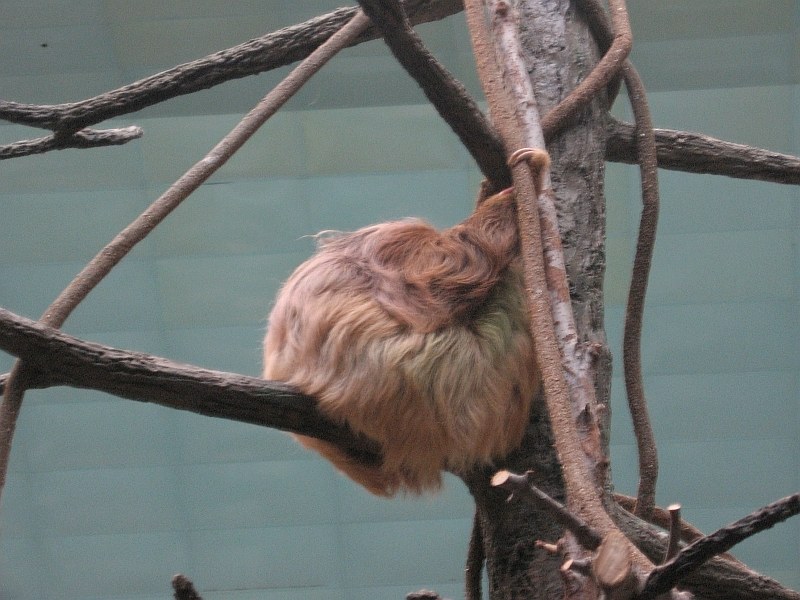This vibrant daytime photograph, likely taken at a zoo, prominently features a small, brown sloth nestled in a leafless tree. The sloth, characterized by its brown fur—ranging from light to dark shades—and long claws, is tightly curled into a protective ball, with one arm wrapped securely around a slender tree branch. The tree's branches, some of which show clean cuts suggestive of saw marks, extend vertically and horizontally, creating a network around the central trunk. In the background, a segmented wall, painted in shades of blue, gray, and green to mimic bricks, stands under the warm sunlight, casting gentle highlights on the scene. The sloth’s compact, ball-like form gives it an almost toupee-like appearance, blending harmoniously with the tree’s natural structure.